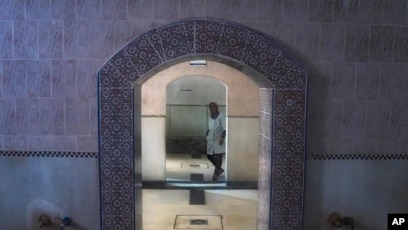The indoor photo depicts a complex, intricately designed scene within a building, showcasing a series of arched doorways. The primary focus is a doorway in the foreground adorned with pink and circular patterned tiles, which frames a subsequent, lighter doorway lined with diverse tile designs. This latter entryway has a more subdued palette with white and light grayish-blue stones and a white base. The visual corridor through these doorways leads to a separate room where a woman stands, clad in a long white coat and black headscarf and pants. The walls inside feature a mix of light pink with white tiles, while the floor is marked by a distinctive white surface containing a solitary black square. In the bottom right corner of the image, the letters "AP" are faintly visible. The image captures the essence of a layered, finely detailed architectural setting, rich in textures and subtle color variations.